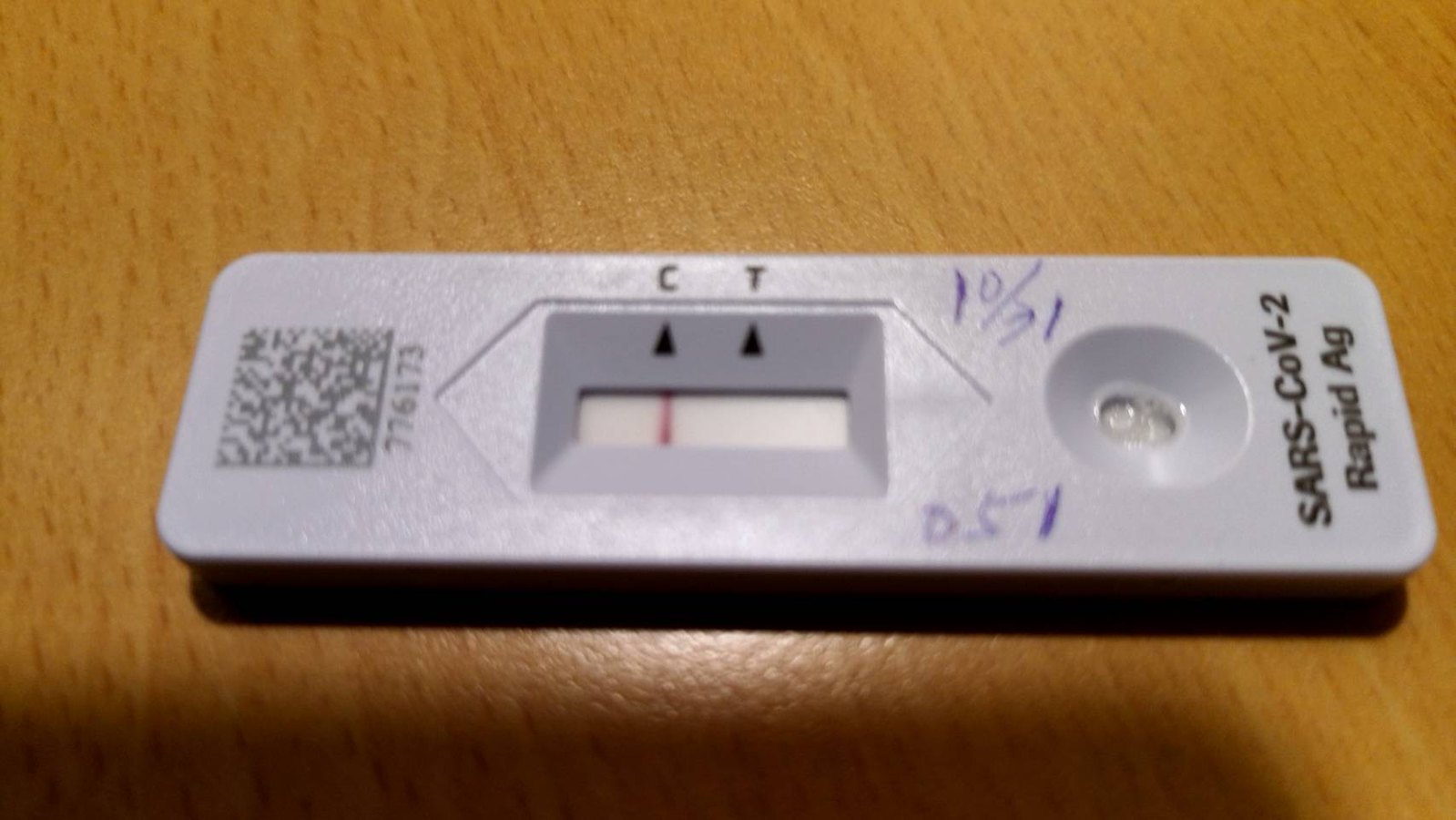The image depicts a horizontally oriented COVID-19 rapid antigen test lying on a tan-colored wooden surface. At the bottom right of the test, the words "SARS-COVID-2" are clearly visible, with "Rapid AG" written below. There is blue handwriting at the top (aligned horizontally) that reads "10-31," and more blue digits "0-5-1," slightly out of focus, are written at the bottom from this angle. The test appears to have been properly administered, with visible saliva in the receptacle. A red stripe is present under the "C" (Control) tab, indicating the test's validity, while no line is visible under the "T" (Test) tab, confirming a negative result. A barcode is located on the top-left side, with the numbers "7-7-6-1-7-3" displayed below it.